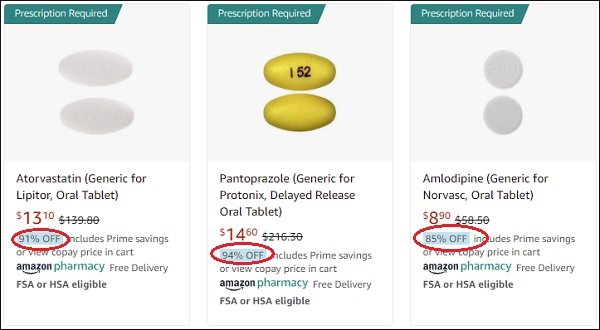This image is a composite screenshot from Amazon Pharmacy, showcasing a comparison of various medications side by side. Each of the three sections displays a different prescription-required medication in a green box at the top. 

- **Left Section:** Features a tan, oval-shaped pill labeled as Atorvastatin, the generic version of Lipitor. It is priced at $13.10 with a highlighted discount of 91% off, circled in red. 
- **Middle Section:** Shows a yellow, oval pill inscribed with "I-5-2", identified as Pantoprazole, the generic version of Protonix in delayed-release oral tablet form. It is offered at $14.60 with a 94% discount, also circled in red. 
- **Right Section:** Displays a dark gray, circular tablet labeled as Amlodipine, the generic version of Norvasc. This medication is priced at $8.90 with an 85% discount, circled in red.

All medications are advertised as being available through Amazon Pharmacy with the benefit of free delivery. The overall image compares the medications’ appearances, purposes, and the significant discounts available on their prices.